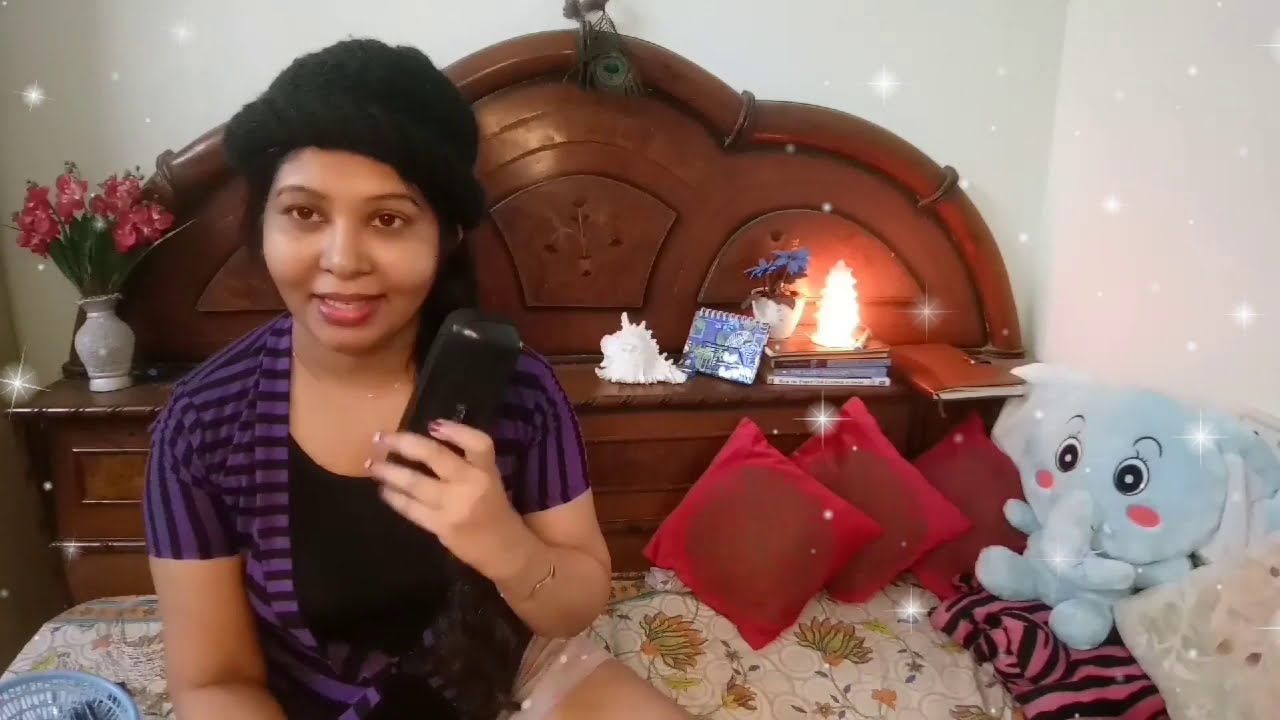The image depicts a young Southeast Asian or Southern Asian woman, likely in her early 20s, sitting on a bed in what appears to be a bedroom. She has medium-toned skin and dark black hair, and she is wearing a black knitted hat. Her outfit consists of a black t-shirt layered under a short-sleeved, purple and black striped shirt that is either tied or buttoned in the middle. She is also wearing tan shorts and has polished nails. A bracelet adorns her left wrist, which is holding a black rectangular case or phone near her head as if she's speaking into it or using it as a Bluetooth speaker. 

The background features a wooden headboard with a ledge, which has a curved, cloverleaf-like design. On the ledge rests a vase with pink flowers, a white seashell, a little lamp, a flip calendar, some books, and possibly a glowing decorative tree. To her right, there are multiple pillows, including red square ones, along with a blue stuffed elephant, atop a striped blanket and a floral print bedspread. The walls behind her are white or off-white. The image appears to have an applied filter, as there are white star effects sprinkled throughout, giving it a sparkling appearance.